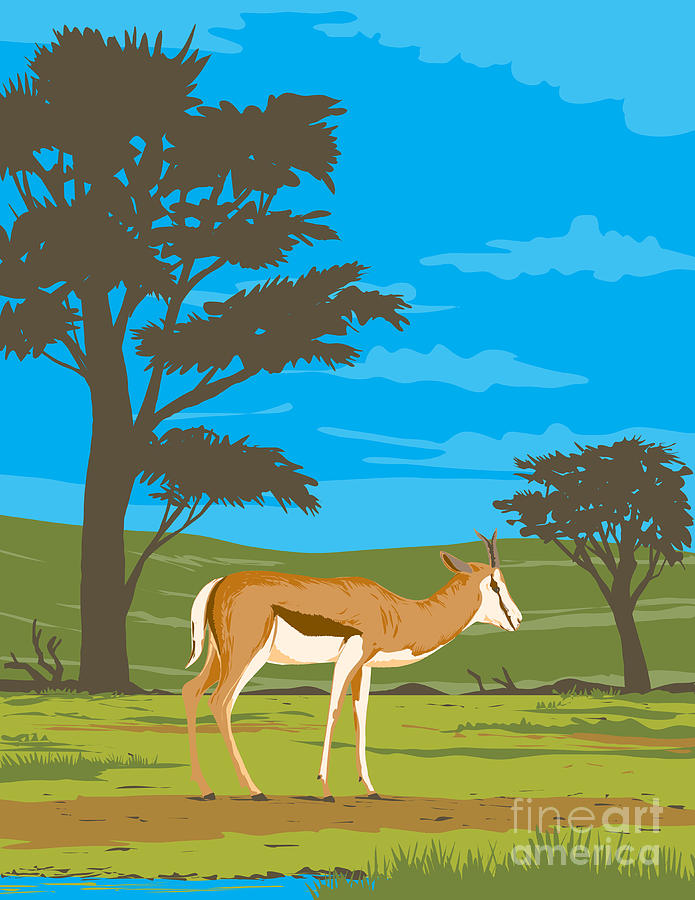This detailed illustration features a stunningly bright, deep blue sky adorned with light blue clouds. Dominating the top half of the image, the sky transitions downward into a lush, olive green hillside, accented with various shades of moss greens to add depth to the terrain. In the foreground, the landscape shifts into a plain with golden-green tones interspersed with patches of brown, suggesting a mix of grass and earth. A blue river meanders on the bottom left, accompanied by green reeds. 

Foreground details reveal an animal resembling an impala or small antelope situated in the middle of the image, facing right. The animal boasts a light tan body with a cream-colored face and underbelly, complete with a white tail and legs. Distinctive features include two horns atop its head, a notable black stripe down the side of its face, and black eyes. Two silhouetted trees, one tall on the left and a shorter one on the right, both shaded in brown, frame the scene. At the bottom right-hand corner, a watermark reads "Fine Art America" in light gray text, adding an artistic touch. The overall setting evokes a serene, possibly African landscape complete with various natural elements.